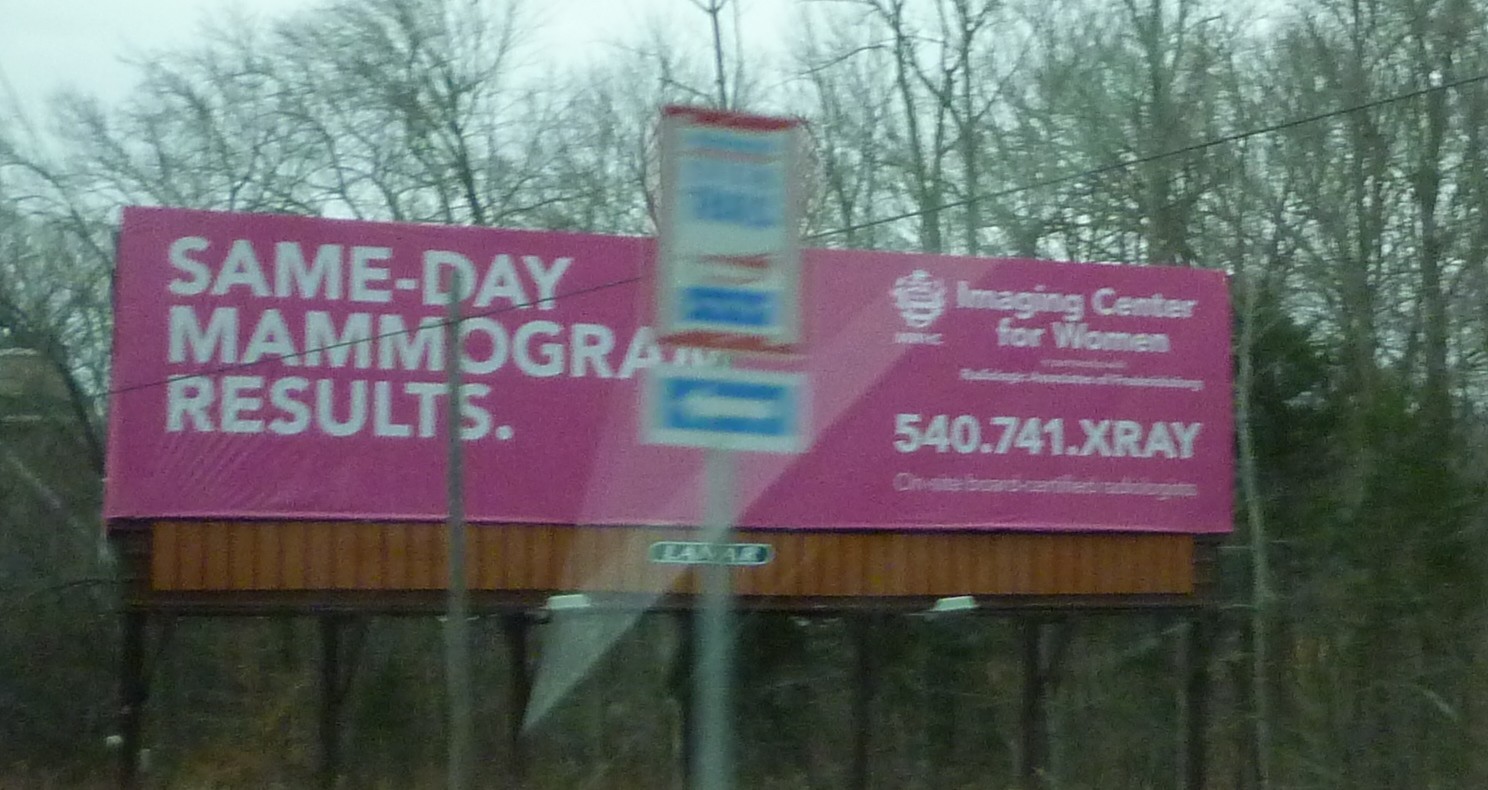The photograph captures a large pink billboard promoting same-day mammogram results, likely taken from a moving car. The image bears the characteristic shadow seen when photographing through a window. The billboard stands out against a backdrop of numerous leafless trees, suggesting it is autumn or winter. In crisp, bold white letters, the billboard advertises “Same-Day Mammogram Results.” To the right, there’s an emblem accompanied by the text "Imaging Centre for Women" and a contact number: 540.741.XRAY. In the foreground, a directional sign with an arrow pointing to the left is visible, although its text is blurred and unreadable. The barren trees in the background add to the overall stark, wintry atmosphere of the scene.